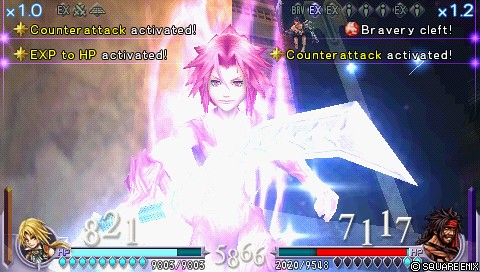This image appears to be a screenshot captured from a video game. Dominating the center is a detailed and somewhat realistic illustration of a woman’s face. She has striking lavender-purple hair. To one side of her, there seems to be what resembles a wing, though it is unclear whether it's part of her or an element from the background. 

At the bottom right corner, there is an icon depicting a soldier—a man wearing a helmet. Adjacent to this icon is the number "7117" displayed in white. On the lower left side, another small icon or avatar is visible, representing a man with long blonde hair. 

In the upper right corner of the image, the words "Bravery Cleft" are prominently displayed, and just below that, the phrase "Counter Attack Activated" can be seen.